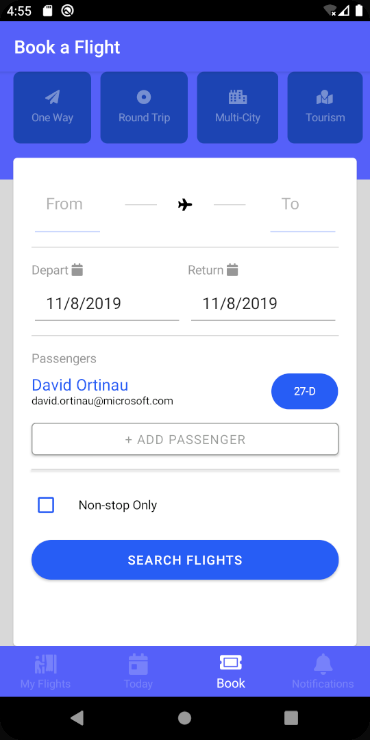The image displayed on the phone screen is predominantly blue and white, featuring an app interface labeled "Book of Light" at the top. The time in the upper left corner is 4:55, accompanied by two small icons, one square and one circular. On the right side of the screen, a Wi-Fi signal icon is crossed out, indicating no available connection, alongside the signal and battery icons.

"Book of Light" is prominently written in white within the blue top section. Below it, there are navigational tabs labeled "One Way," "Round Trip," "Multi-City," and "Tourism." The user has selected the screen where travel details are entered. It shows fields for "From" and "To" with a small airplane icon between them. The departure and return dates are both set to 11-8-2019.

Passenger details include the name David Artineau and his email, davidartineau@microsoft.com. David has been assigned seat 27D. There is an option to add another passenger via a plus sign, and a checkbox for "Non-Stop Only" flights. A prominent blue "Search Flights" button is available for initiating the search.

At the very bottom of the screen are navigation icons labeled "My Flight," "Today," "Book," and "Notifications." The "Book" icon is currently highlighted, indicating the active section of the app.